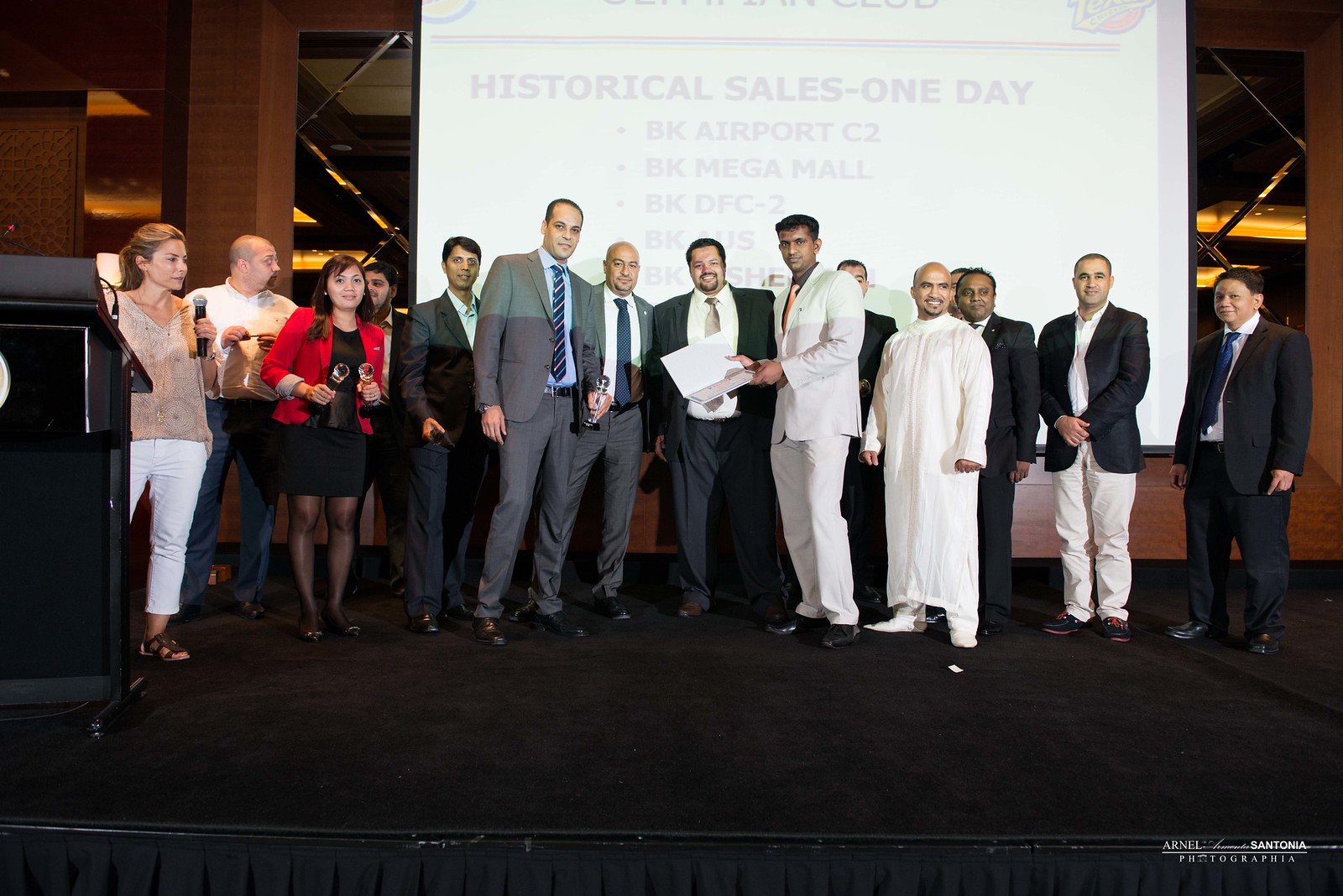The photograph captures a vibrant and detailed scene on a brightly-lit stage where fifteen people are posed together, celebrating an evident achievement. The majority of individuals are men dressed in business suits, while a few women stand to the left, with one holding a microphone and another in a red jacket displaying two awards. All are smiling at the camera, conveying a sense of pride and accomplishment.

In the background, a projector screen prominently displays the words "Historical Sales One Day," along with a partially obscured list that includes locations like BK Airport C2, BK Mega Mall, BK DFC-2, BK AUS, and BK SHE. At the center of the group, a man in a long white robe stands out, holding an open certificate, emblematic of their achievement.

The stage is adorned with a black skirt, and a podium is positioned on the left. The bottom right-hand corner of the image is marked with the photographer's credit, "Arnel Santonia Fotografia." The image is clear and colorful, capturing the celebratory atmosphere of the moment.